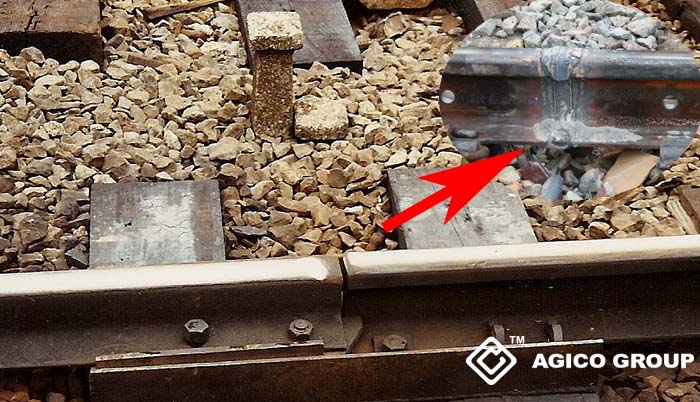The image showcases a close-up view of railroad tracks outdoors. The tracks are bordered by steel beams with large bolts. In between the rails, there are numerous small stones. Wooden planks are partially visible, crossing beneath the stones but cut off squarely. In the top right corner, a circular or oval overlay zooms in on the track rails being welded together, marked by a red arrow. This inset provides a different angle, showing some weathering on the steel beams. Additionally, a logo featuring a diamond within a diamond and the text "AG ICO group" appears at the bottom of the image.